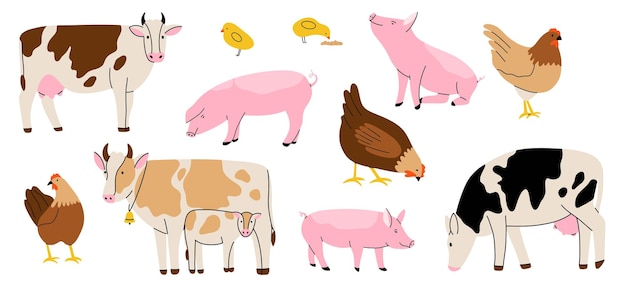In this cartoon drawing of an array of farm animals, we see a variety of creatures, each depicted with charming detail. In the upper left corner, there is a brown and white Holstein cow with little horns, a pink udder, a pink ear, and a pink nose. Surrounding the cow, there are yellow chicks, one of which is bending down to peck at some yellow grains. Below this scene, a bright pink pig is walking around, while another pig, also pink, is sitting on its haunches with its nose in the air.

To the right of the standing pig, another cow grazes, its head down, showing off a pink udder. This cow has a black and white body. Above this grazing cow, in the right corner, stands a brown and white hen with a red comb and tan feathers. Another pig is seen between this hen and the grazing cow. Further to the right is another cow, adorned with a bell around its neck, accompanied by a calf. Additional small details include another hen with brown feathers and a little light tan around its neck.

Overall, the image vividly showcases a bustling farm scene with cows, pigs, hens, and chicks, each performing their endearing, everyday activities.